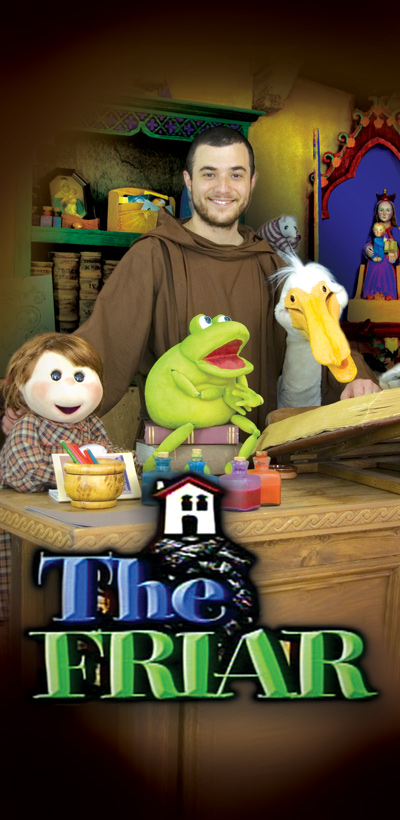The image appears to be a promotional photograph for a children's puppet show titled "The Friar." Dominating the center of the photo is a young, white man with black hair, a dark beard, and a warm smile, dressed in a brown hooded monk's robe. He is standing at a workshop table cluttered with a variety of puppets and toys. The table includes a green frog puppet resembling Kermit the Frog, which has an open mouth revealing a red interior, perched on a stack of books. To the frog’s left is a white pelican puppet with a bright yellow beak. To the frog's right is a human-like boy puppet with brown hair, wearing a flannel shirt; the man touches its shoulder affectionately. 

Behind this lively scene, the backdrop is a vibrant and colorful puppet theater set, featuring shades of green, red, orange, and yellow, giving the setting a playful and engaging atmosphere. Additional details include a green shelf hovering above the man’s head, holding various items, possibly toys or workshop tools, with some brown stacks and framed artwork—a likely depiction of Mary and baby Jesus—adding to the background's complexity. 

The lower part of the image showcases the logo for the show. The logo features the words "The Friar," with 'The' in blue and 'Friar' in green, both superimposed over an illustration of a small white cottage with a red roof, black windows, and a black door, resting on what appears to be a black rock foundation. This descriptive and visually enriching scene sets a captivating tone for the children's show it promotes.